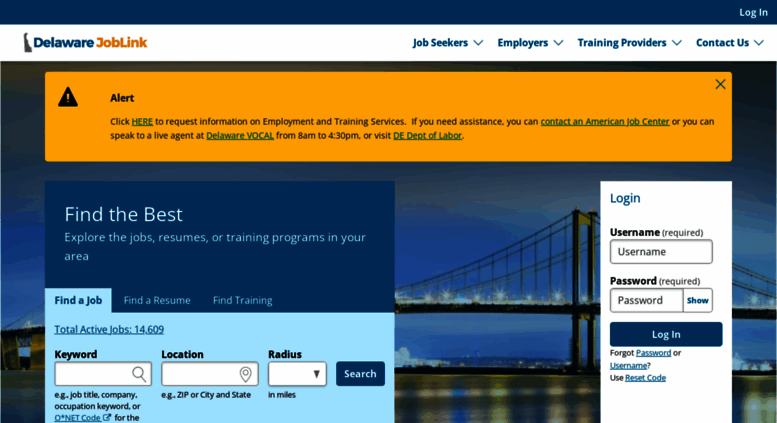The illustrated webpage is from the Delaware JobLink website. The site prominently features an image of the state of Delaware, colored in blue, with the text "JobLink" highlighted in yellow. In the top navigation bar, options available to users include: "Job Seekers," "Employers," "Training Providers," and "Contact Us."

An alert is immediately noticeable; a yellow banner with a black triangle containing a yellow exclamation point. The alert message reads: "Click here to request information on employment and training services. If you need assistance, you can contact an American Job Center or speak to a live agent at Delaware Local or VOCAL from 8 a.m. to 4:30 p.m. You can also visit the Delaware Department of Labor."

Below the alert, the webpage encourages users to "Find the Best" by exploring job listings, resumes, and training programs available in their area. Clear action buttons labeled "Find a Job," "Find a Resume," and "Find Training" guide users to their respective searches.

Further down, a login section requires users to enter a username and password, with both fields marked as required. Users have the option to display their password by clicking "Show." The "Log In" button is conspicuously in teal color.